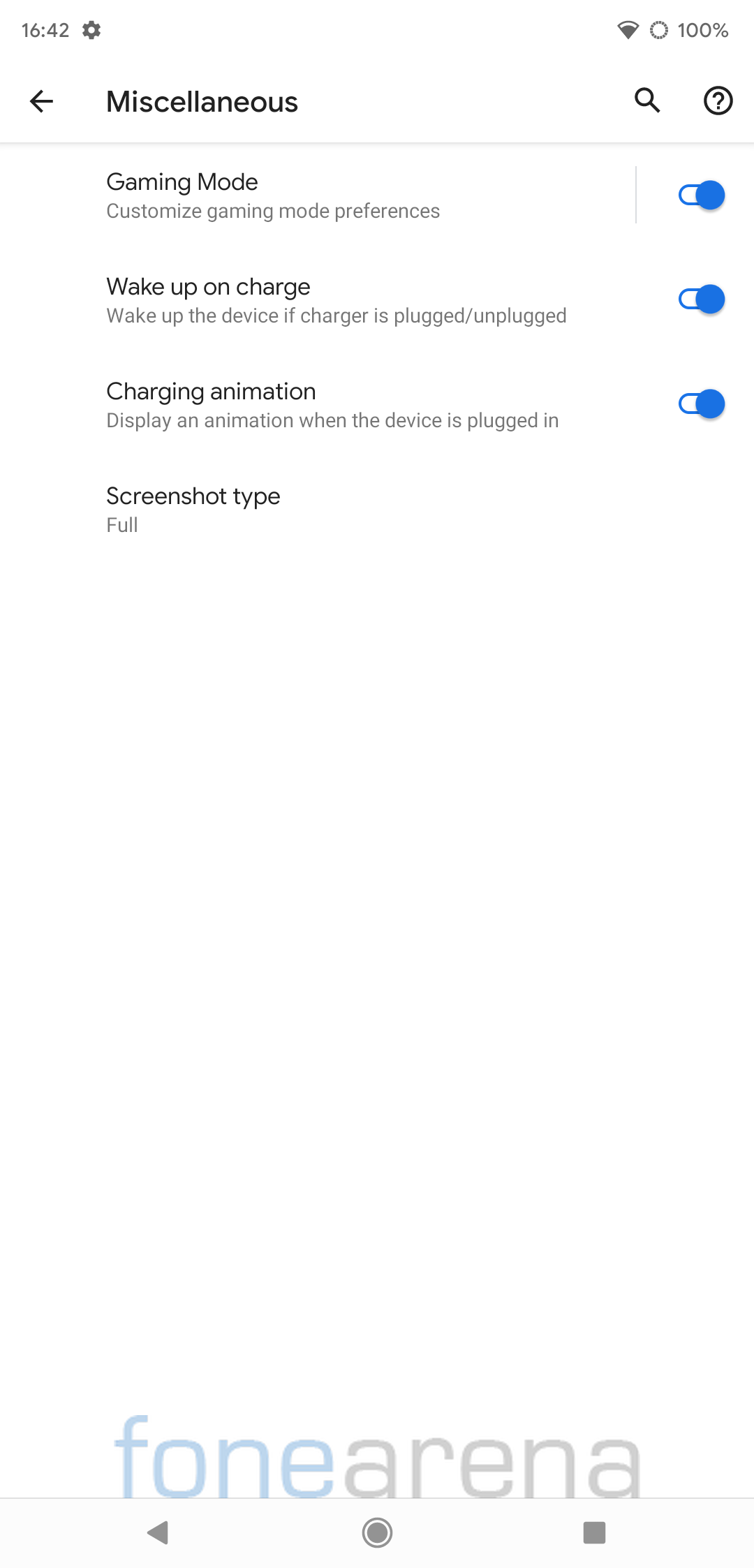Here is a cleaned-up and detailed caption for the image described:

---

This screenshot from a mobile device displays a settings menu with several key features. At the bottom of the screen are navigation icons – back, home, and tabs – in gray on a white background. Above this is a watermark reading "fonearena," with "fone" in blue and "arena" in gray. The time is displayed at the top of the screen, showing 16:42, along with a settings cogwheel icon, a Wi-Fi indicator, and a fully charged battery symbol (100%) in the upper right corner.

The main content area starts with a back arrow pointing left, followed by the word "Miscellaneous" in bold black font. To the right, there are search and help icons. Below this section, various settings are listed, including "Gaming Mode," "Customized Gaming Mode Preferences," "Wake Up on Charge" (which wakes the device if the charger is plugged or unplugged), and "Charging Animation" (that displays an animation when the device is plugged in). The setting "Screenshot Type" is indicated as "Full." The top three options are all enabled, as shown by blue toggle switches on the side, indicating that these features are turned on.